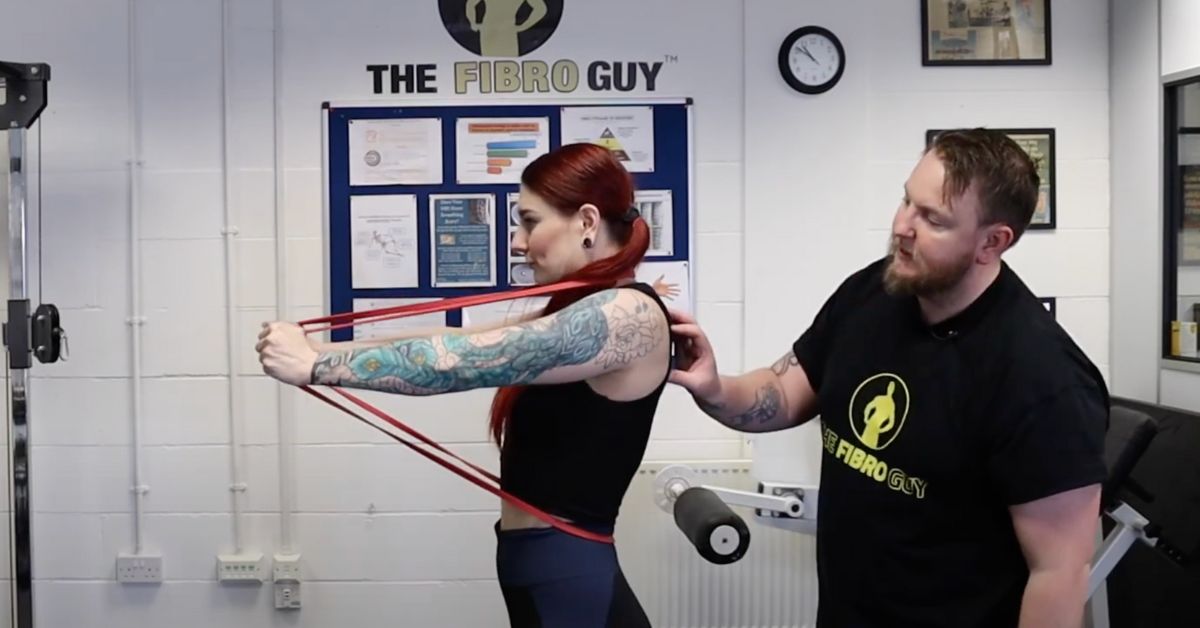In the image, a woman with long, bright red hair tied in a ponytail is working out in a gym. She is wearing a black tank top and blue workout pants. Her left arm is adorned with a detailed full-sleeve tattoo featuring a blue snake and possibly other elements, extending from her wrist to her shoulder. She is in the middle of an exercise, stretching a red resistance band in front of her, which is looped around her waist and neck. Behind her stands a man with short brown hair and a brown beard, wearing a black t-shirt emblazoned with "The Fibro Guy" in yellow letters—the same logo is also visible on the back wall, emphasizing that this is likely his brand. The man has his right hand placed on her back as though assisting or guiding her, his fingers splayed outward. The backdrop of the gym features various workout equipment, including a leg machine and a weight pulley, reinforcing the active environment.